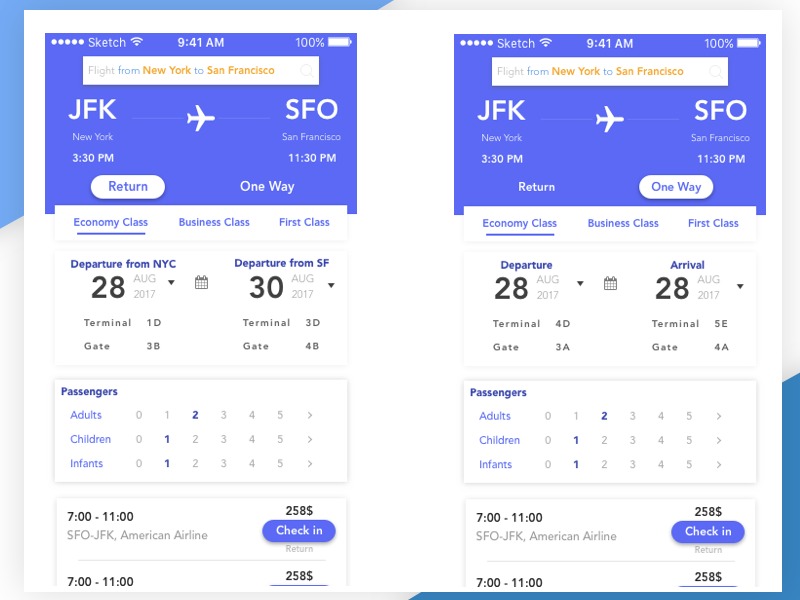This is a detailed and descriptive caption for the screenshot provided:

---

A screenshot displays two flight options side-by-side, featuring a unified white background with purplish-blue headers occupying the top third of each section. Each option presents a set of slightly varied details in a similar layout. 

In the left section, a search bar at the top reads "Flight from New York to San Francisco" with both "New York" and "San Francisco" highlighted in mustard yellow. Below the search bar, flight details are provided: 
- Departure from JFK, New York at 3:30 PM.
- An icon of an airplane is positioned above a thin white line.
- Arrival at SFO, San Francisco at 11:30 PM.

Beneath these details, two buttons are displayed:
- "Return" is in purple text enclosed in a white pill-shaped border.
- "One Way" is written in white text without any border.

Following the buttons, three travel class options are listed on a white rectangular background:
- "Economy Class," which is underlined.
- "Business Class."
- "First Class."

Below the class options, another rectangular section contains the flight details and departure information:
- On the left: "Departure from NYC, 28 August 2017" with a downward arrow and a calendar icon in the middle.
- On the right: "Departure from SF, 30 August 2017" with a downward arrow.

Further down, terminal and gate details are provided:
- On the left: "Terminal 1D, Gate 3B."
- On the right: "Terminal 3D, Gate 4B."

At the bottom, a rectangle outlines passenger details with categories listed below it:
- "Passengers."
- Followed by "Adults," "Children," and "Infants."

The screenshot organises flight information in a clear and structured manner, facilitating easy comparison between the two options.

---